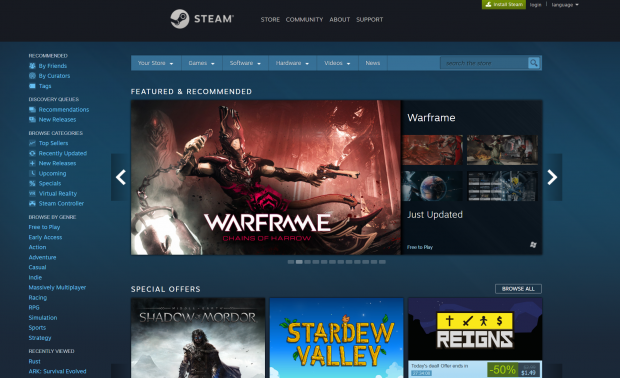This image captures the vibrant homepage of the Steam online gaming store. At the top of the page, the iconic Steam logo is prominently displayed alongside key navigation options: Store, Community, About, and Support. In the upper right-hand corner, users can log in to their accounts, change the language settings, and see their profile names highlighted in green lettering.

The left-hand sidebar offers a well-organized menu for game selection, including categories like Recommended, Discovery, Browse Categories, Browse by Genre, and Recently Viewed Games. 

Dominating the middle section of the page are dynamic visual previews of various games. The first featured game is "Warframe," with navigation arrows allowing users to browse through other game options. Below this showcase are additional game titles, including "Middle-earth: Shadow of Mordor," "Stardew Valley," and "Reigns." 

An area dedicated to special offers entices users to explore current deals further. The main navigation menu features tabs for Store, Genres, Software, Hardware, Videos, and News. This comprehensive and user-friendly layout ensures an engaging and efficient browsing experience for gamers.